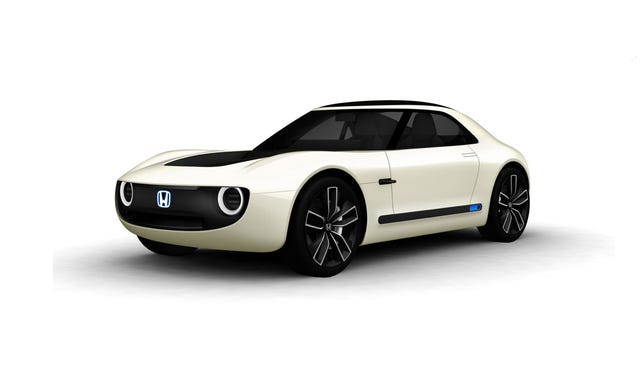This image showcases a sleek, modern Honda EV concept car, positioned at about a 30 to 45-degree angle, accentuating its driver's side and front. The car's sophisticated design features a predominantly white body with a striking black hood, roof, and grille. A black stripe runs along the door, culminating in a distinctive blue rectangle near the rear. The vehicle sports tinted black windows, including a sunroof. The illuminated Honda 'H' logo stands prominently on the front bumper, framed by circular black-filled headlights. The car boasts black and silver rims with a five-spoke design and an integrated Honda logo. The setting is minimalist with a solid white background and floor, ensuring the car's details are the focal point. This two-door car, reminiscent of a sports car, exudes a hybrid or electric vibe, enhancing its futuristic appeal.